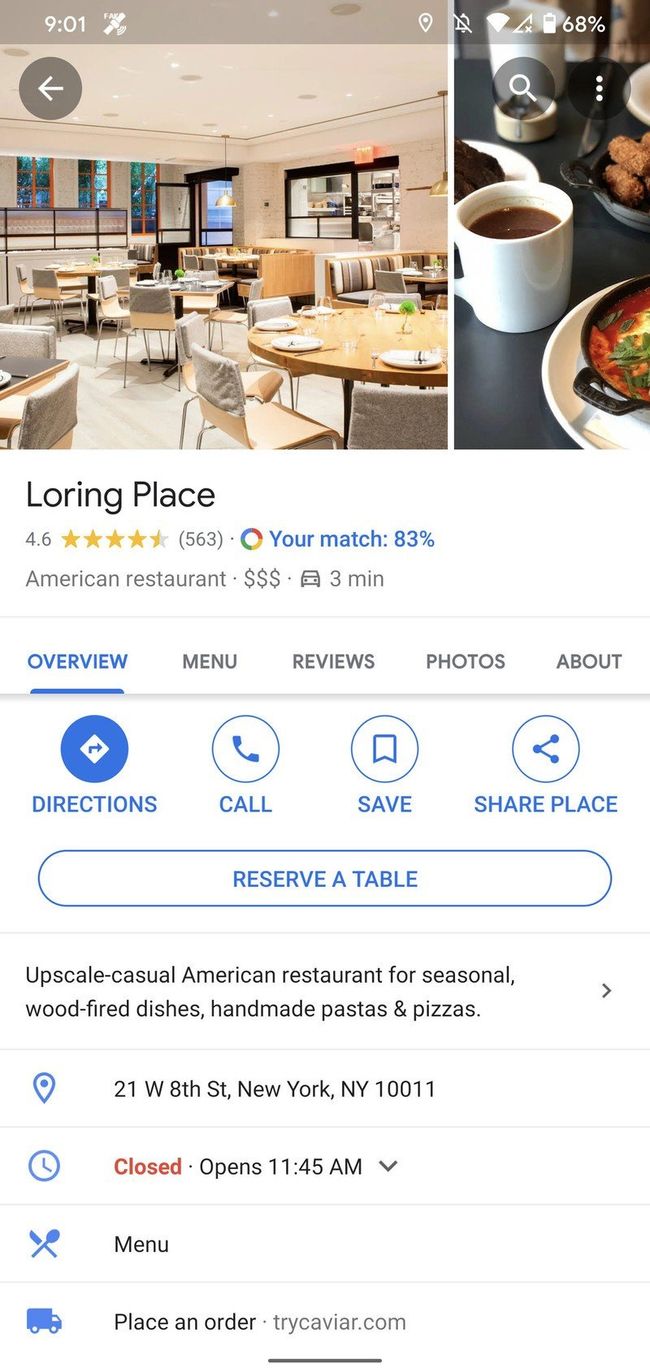Screenshot of a cellphone display featuring various details. At the top of the screen, there's a grey bar overlaying a background image. The white text within the bar shows the time as 9:01, followed by an unfamiliar symbol resembling a space satellite, with some illegible small text next to it on the upper left. On the right side of the bar, there are GPS coordinates, indicating that sound is off, full WiFi strength, no cell coverage, a mostly full battery with the percentage shown as 68%. 

Below this, the screen displays an image of a tastefully designed modern restaurant or cafe, with white flooring, white chairs, and tan wooden tables. To the right, there's a white cup filled with a dark liquid, presumably coffee. Underneath the image, in black text, the name "Warren Place" is displayed, with a rating of 4.6 stars. It states that your match score for this place is 83%, highlighted in blue.

Beneath this, a blue underlined "Overview" is listed, followed by menu options in black text: "Menu", "Reviews", "Photos." Additional options like "Directions", "Call", "Save", "Share Place", and "Reserve a Table" are shown, with the last three being in black. The restaurant is described as an "upscale, casual restaurant for seasonal wood-fired dishes, handmade pastas, and pizzas" located at "21 West 8th Street, New York, NY". It is currently closed and will reopen at 11:45 AM. 

A blue bar at the bottom of the display provides options to view the menu and place an order. This marks the conclusion of the current content on the screen, ready to proceed to the next item.